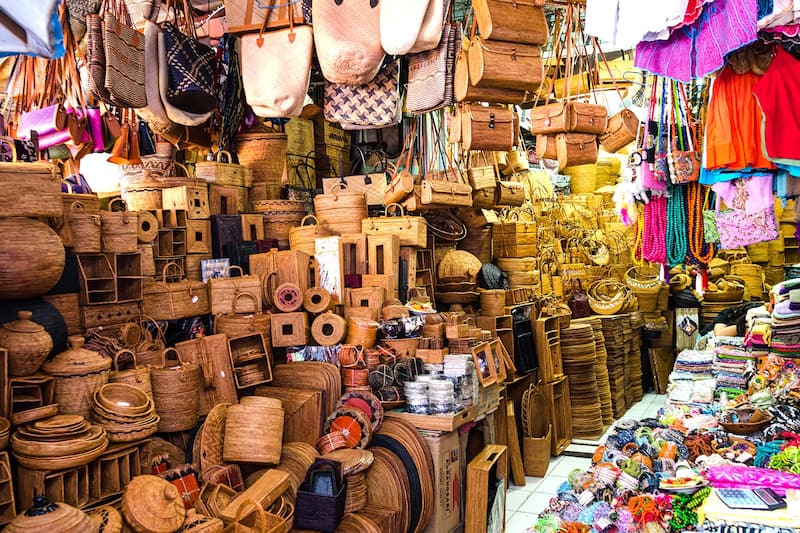This full-color horizontal photograph showcases an intricately packed indoor market store, illuminated naturally. The left side of the image features an extensive assortment of brown, wooden, and woven objects, including baskets, boxes, and barrels. These items are either hanging, placed on shelves, or stacked on the floor. Above these are numerous handbags and purses, varying in shades from white, brown, and black, to light pink and dark blue. Some of these handbags seem designed for specific uses, such as carrying cases for binoculars. 

Transitioning to the center right, the image highlights a clutter of gold baskets and boxes, arranged amidst the brown objects, adding a touch of metallic contrast. Moving further right, there is a table covered with a profusion of colorful fabric objects, likely including clothes and accessories, though their exact nature is not entirely clear. Above this vibrant area, additional fabric items such as women's bags, clothing in purples, reds, and oranges, and possibly children's garments hang from the ceiling. 

In the lower right corner, a collection of multi-colored necklaces and trinkets add to the decorative assortment. The scene is completed by a narrow pathway, allowing for navigation through this densely adorned market space.